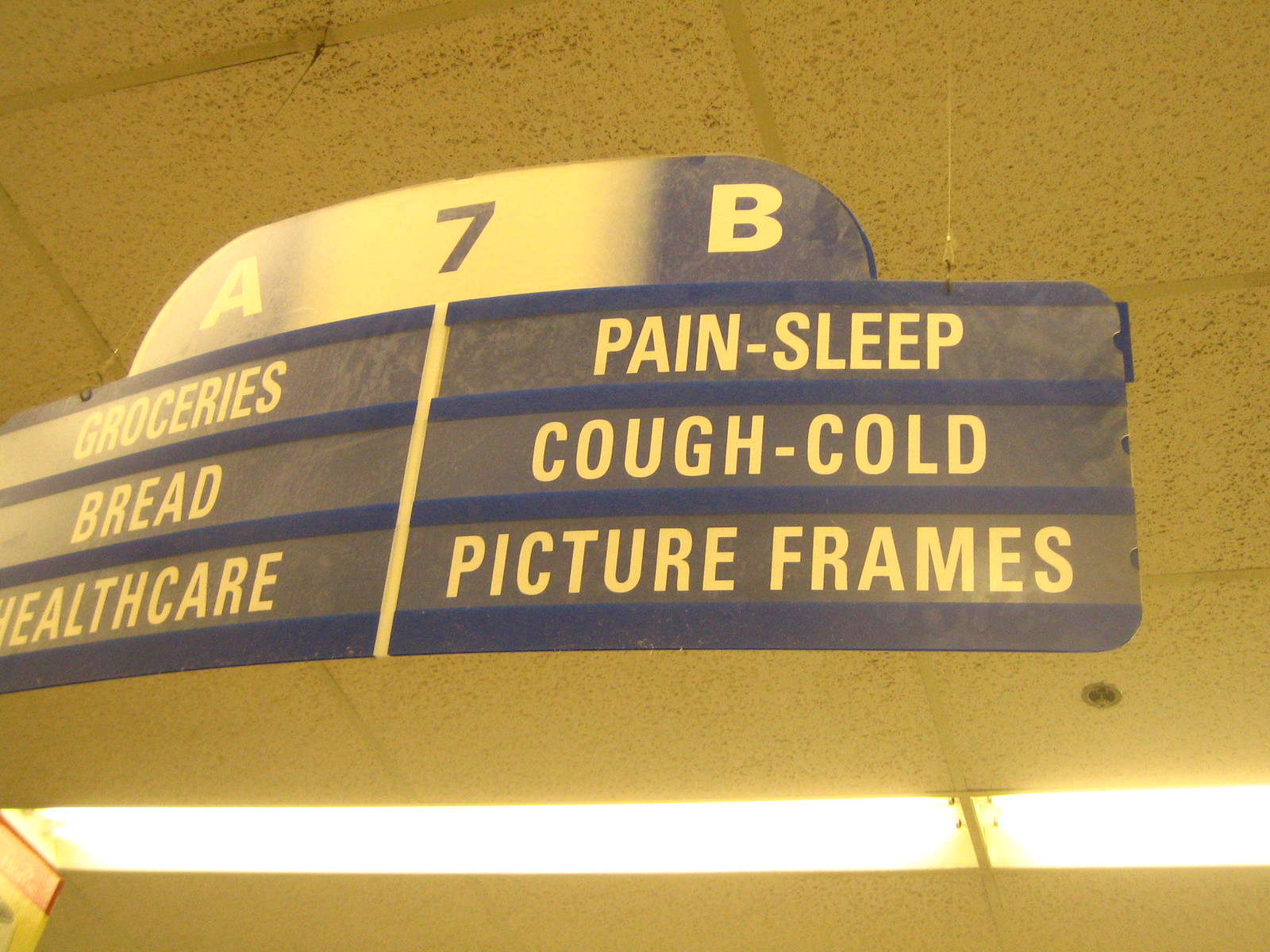The image depicts a well-lit supermarket aisle with a sign marker hanging from the ceiling, indicating aisle 7. The ceiling has white, speckled panels with bright fluorescent lights. The aisle marker is blue, featuring a large number "7" prominently in the center. The sign is divided into two sections: on the left side (labeled 'A'), in bold, white uppercase letters, it lists "GROCERIES," "BREAD," and "HEALTHCARE." On the right side (labeled 'B'), it details "PAIN-SLEEP," "COUGH-COLD," and "PICTURE FRAMES." Additionally, a beige towel with horizontal and vertical lines forming small squares is visible at the bottom of the image.